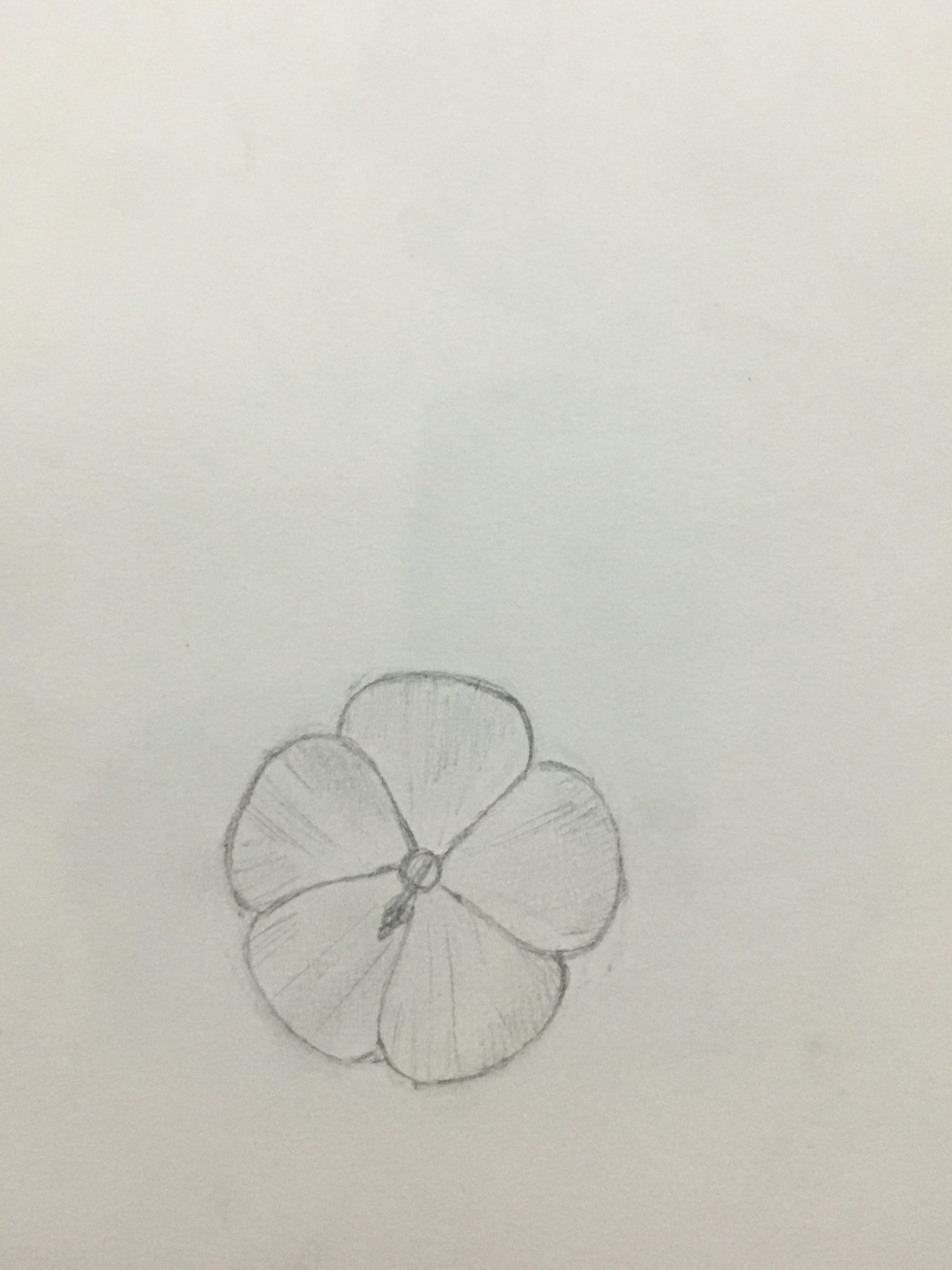This image is a simple yet detailed pencil sketch on plain white paper, positioned on the bottom half of the sheet. The composition features a flower with five petals, each petal having a heart-like silhouette that is lightly shaded to give a textured appearance. The petals radiate around a central stamen, which is extending slightly to the left towards the observer with little poofy parts at the end, suggesting an upward pull as if it's reaching for natural light. The overall effect of the pencil work includes some smudges around the edges, indicating the artist's hand at work. Despite the minimalistic approach, the sketch's careful shading and clear outlines bring the flower to life, making it more advanced than a basic drawing.